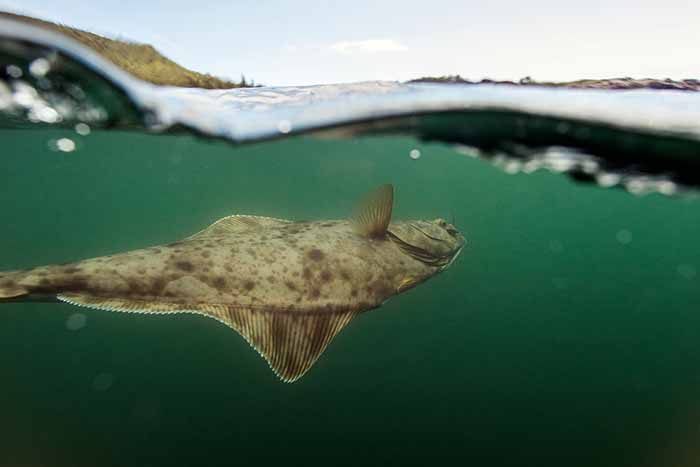This captivating image showcases a serene aquatic scene captured with the camera lens positioned halfway below the water's surface and halfway above. Below the waterline, the murky, greenish aquamarine-colored water gently darkens towards the bottom, creating a mysterious ambiance. The underwater centerpiece is a unique and ancient-looking fish, possibly a flounder, characterized by its dorsal-ventrally flattened body and two eyes on top. The fish is grayish-brown, adorned with speckles and spots, and features prominent fins on both sides as well as a smaller fin near its head. Above the water's surface, the scene transitions to a swampy, grassy bankside, with hints of dead vegetation in the background. The sky above is a blend of blue and white, with clouds diffusing the sunlight, making the right part of the image slightly brighter. The overall effect of the scene blurs the line between water and sky, creating a harmonious blend of nature's elements.